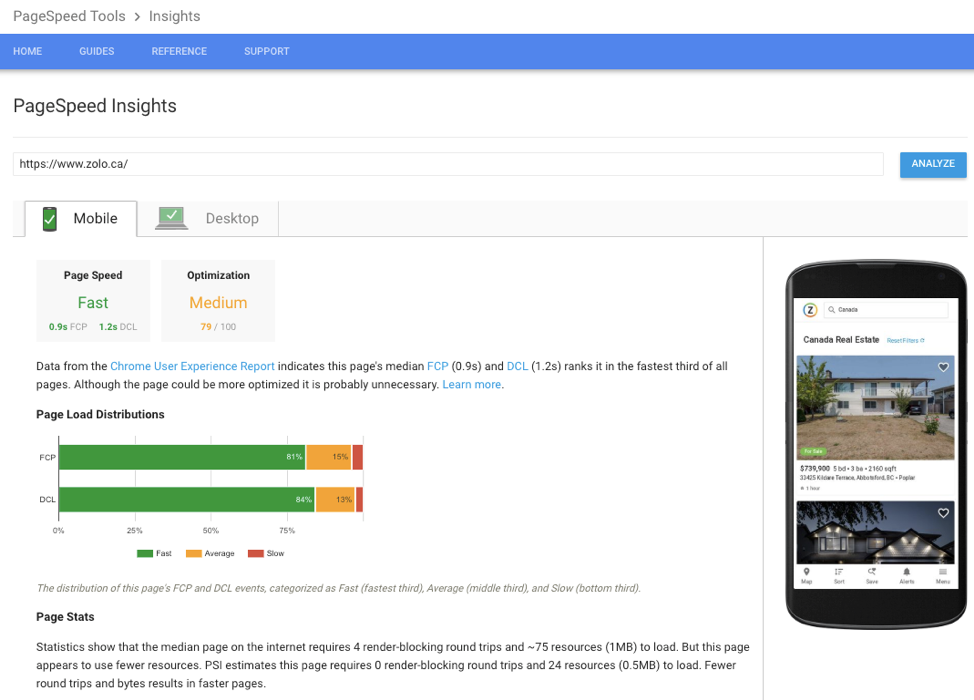Screenshot of the PageSpeed Insights Website

The screenshot captures the PageSpeed Insights webpage. At the top, set against a white background, the text "PageSpeed Tools" appears, followed by a rightward arrow and then the word "Insights." Both "PageSpeed" and "Tools" start with uppercase letters.

Directly below this, a medium blue banner with a hint of purple contains text links for "Home," "Guides," "References," and "Support" in white.

Progressing downward, the page returns to a white background where "PageSpeed Insights" is prominently displayed. The terms "PageSpeed" and "Insights" are written as one word each, both starting with capital letters ("PageSpeed" has a capital 'P' and 'S', while "Insights" has a capital 'I').

Following this header, a web address input field is shown with a prominent blue "Analyze" button featuring white text. Users can choose between mobile and desktop analysis options, with the mobile option currently selected.

The mobile analysis indicates the page is "Fast" with metrics of 0.9 seconds FCP (First Contentful Paint) and 1.2 seconds DCL (DOMContentLoaded). The optimization score stands at 79 out of 100, color-coded in orange to denote its medium status.

Below these metrics, a note states that the data is sourced from the Chrome User Experience Report. The report suggests that the page is deemed medium overall, with FCP at 0.9 seconds and DCL at 1.2 seconds, ranking it in the fastest third of all pages. While the page could be more optimized, it is probably unnecessary.

A "Learn More" link, highlighted in blue with a capital 'L', is provided. Below it, there's a section titled "Page load distributions," featuring a chart categorized into fast, average, and slow. Lastly, a segment entitled "Page Stats" is noted but not detailed in the screenshot.